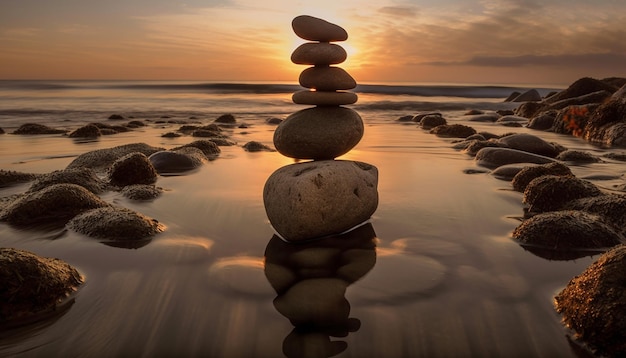The image captures a serene sunrise or sunset scene, characterized by a horizontal, landscape-oriented perspective. At its center stands a meticulously balanced stack of six smooth, flat-ish rocks of varying colors and sizes. The stack begins with an off-white rock at the base and works its way up through various shades of brown, culminating in darker tones at the top. These rocks are positioned at the shallow end of a calm pool of water, which appears to be part of or adjacent to the ocean. Underneath and surrounding the stack, smaller rocks protrude from the shallow water. The sun itself is hidden behind the second rock from the top, casting a warm, radiant glow that transitions from white and yellow at the center to orange, red, and finally to purples and blues as it spreads across the partly cloudy sky. There are paths of rocks leading toward the ocean, where a gentle wave can be seen in the distance. The overall composition and coloration of the sky suggest a peaceful, reflective moment either at dawn or dusk.